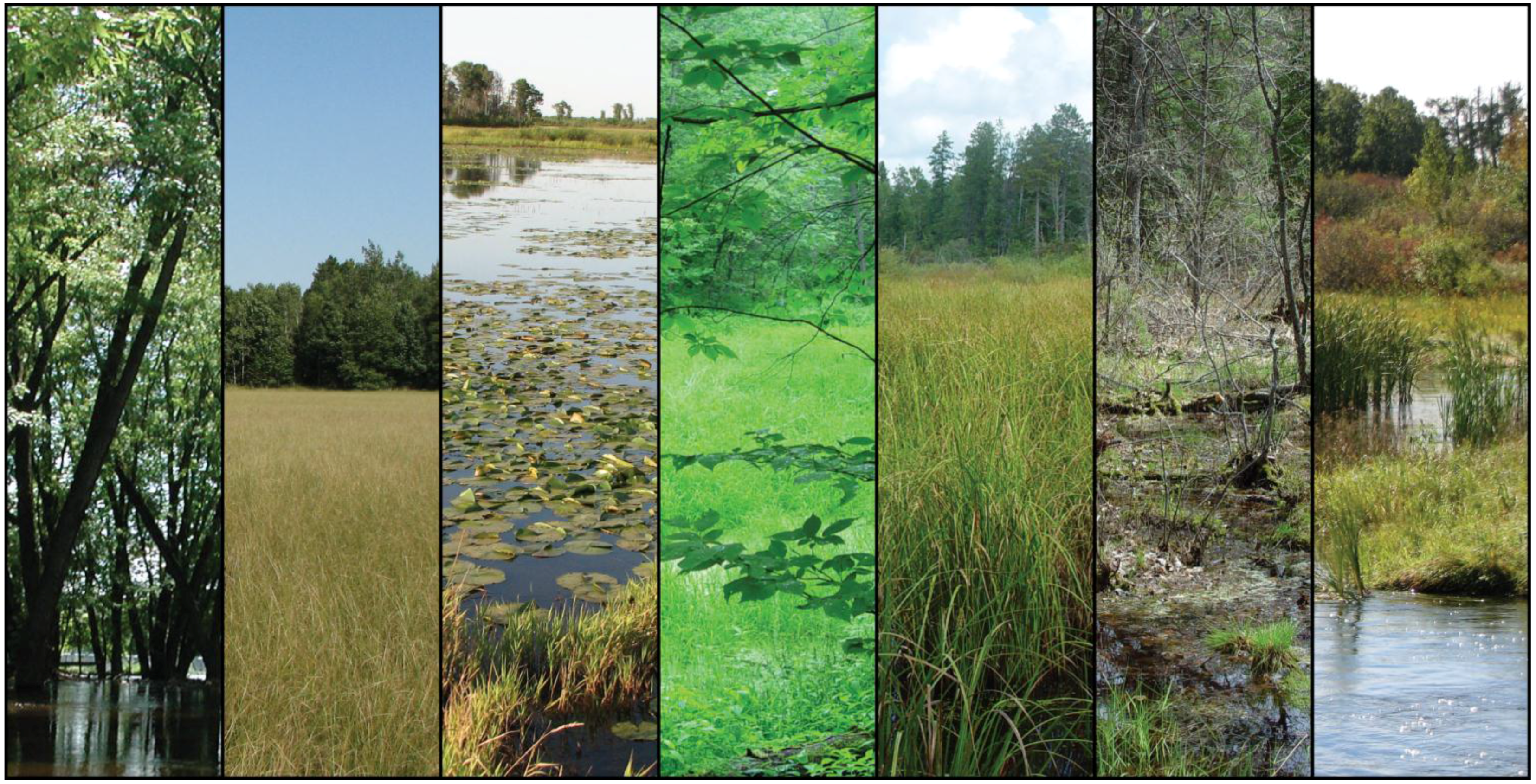A series of seven vertical, rectangular photographs are arranged side-by-side, each encapsulated by a thin black border with black lines separating them. These images, rich in browns and greens, collectively depict various scenes of nature and wilderness, emphasizing the presence of water and vegetation. 

The first photograph shows trees with green leaves growing out of water, their reflections clearly visible below, suggesting a watery environment similar to a mangrove. The second photo captures a vast, open field with tall, greenish-brown grass, bordered in the distance by a line of trees. 

In the third image, there's a pond adorned with lily pads and surrounded by green grass. The fourth photo is more abstract, featuring a dense, lush wooded area with an indistinct green expanse, giving an impression of being deep in a forest. 

The fifth image transitions to a marshy area with tall, weedy grass and evergreen trees in the background. The sixth picture reveals a small brook or stream gently meandering through the woods. 

Finally, the last photograph on the right depicts wetlands or a river with tall grasses on its shoreline, possibly cattails or reeds. The distant tree line is a mix of predominantly green leaves with hints of gold and brown, indicating a transitional season. Together, these images encapsulate the essence of natural landscapes, intertwining elements of forest, water, and open fields.